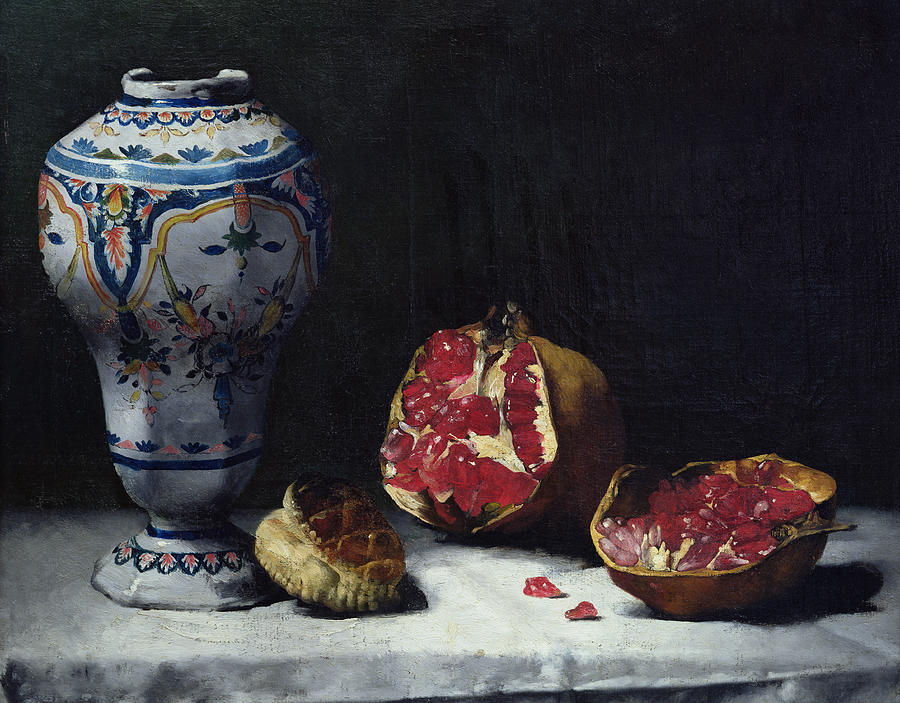The image portrays a detailed still-life painting of a tabletop scene set against a dark background. Central to the composition is an intricately designed vase featuring floral patterns in vibrant hues of blue, white, red, and orange. The vase, larger at the top and tapering towards the bottom, stands prominently on the left side of the pale gray table covered with a white cloth. 

Adjacent to the vase is a large, split open pomegranate, displaying its vivid red and white insides with a brown exterior. The fruit is depicted in halves, one lying flat and the other standing upright, with additional loose seeds scattered around, emphasizing their rich, juicy red color. These elements contribute to the textured complexity of the scene, juxtaposing the sturdy, ornate vase with the organic, segmented pomegranate, creating a visually stimulating tableau.